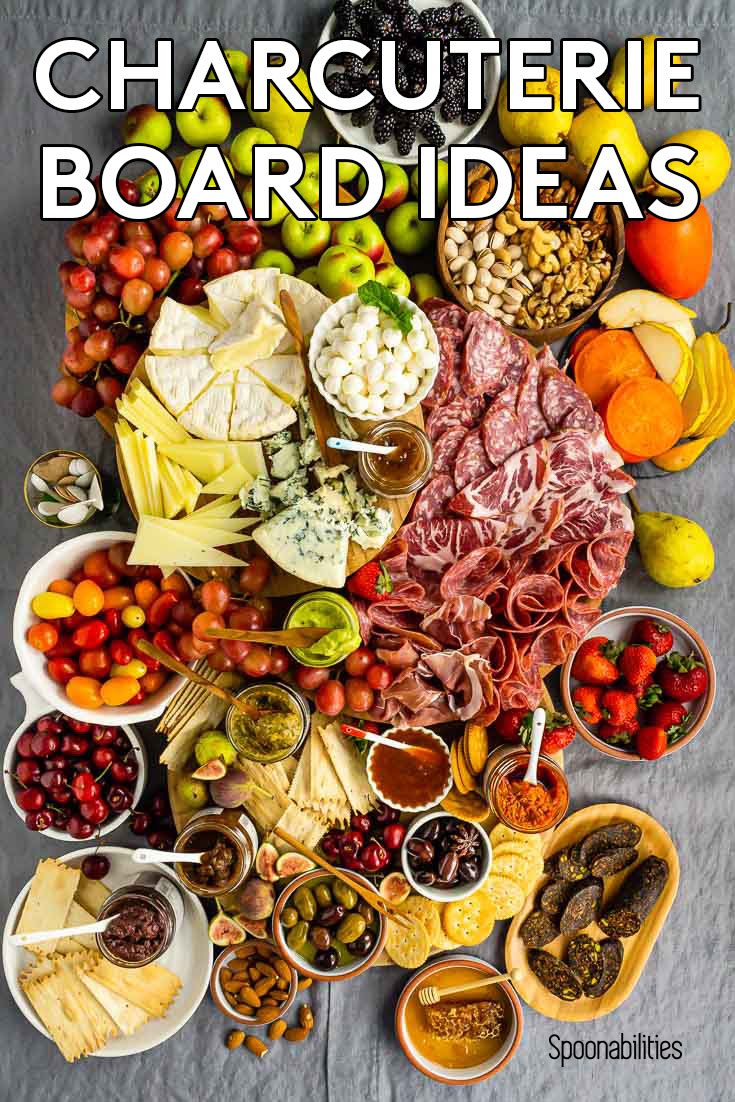This detailed color image showcases a beautifully arranged charcuterie board, presented from an overhead perspective on a gray textured tabletop. Bold white text with a black outline at the top reads "Charcuterie Board Ideas," while in the lower right, black text spells out "Spoonabilities." The arrangement features a large central plate of assorted luncheon meats. To the upper left, a round wooden board displays sliced cheeses and mozzarella balls. At the very top, a white bowl filled with blackberries is surrounded by various nuts, including pistachios, walnuts, and cashews, complemented by a variety of fruits like red grapes, pears, and apples. Below this, another wooden board holds bowls of olives, strawberries, and cherries. In the lower left, a white ceramic plate contains a selection of crackers. Scattered across the gray surface are additional fruits and vegetables, including more apples, squash, tomatoes, and salsas, alongside delicate bowls filled with honey and various other accompaniments.